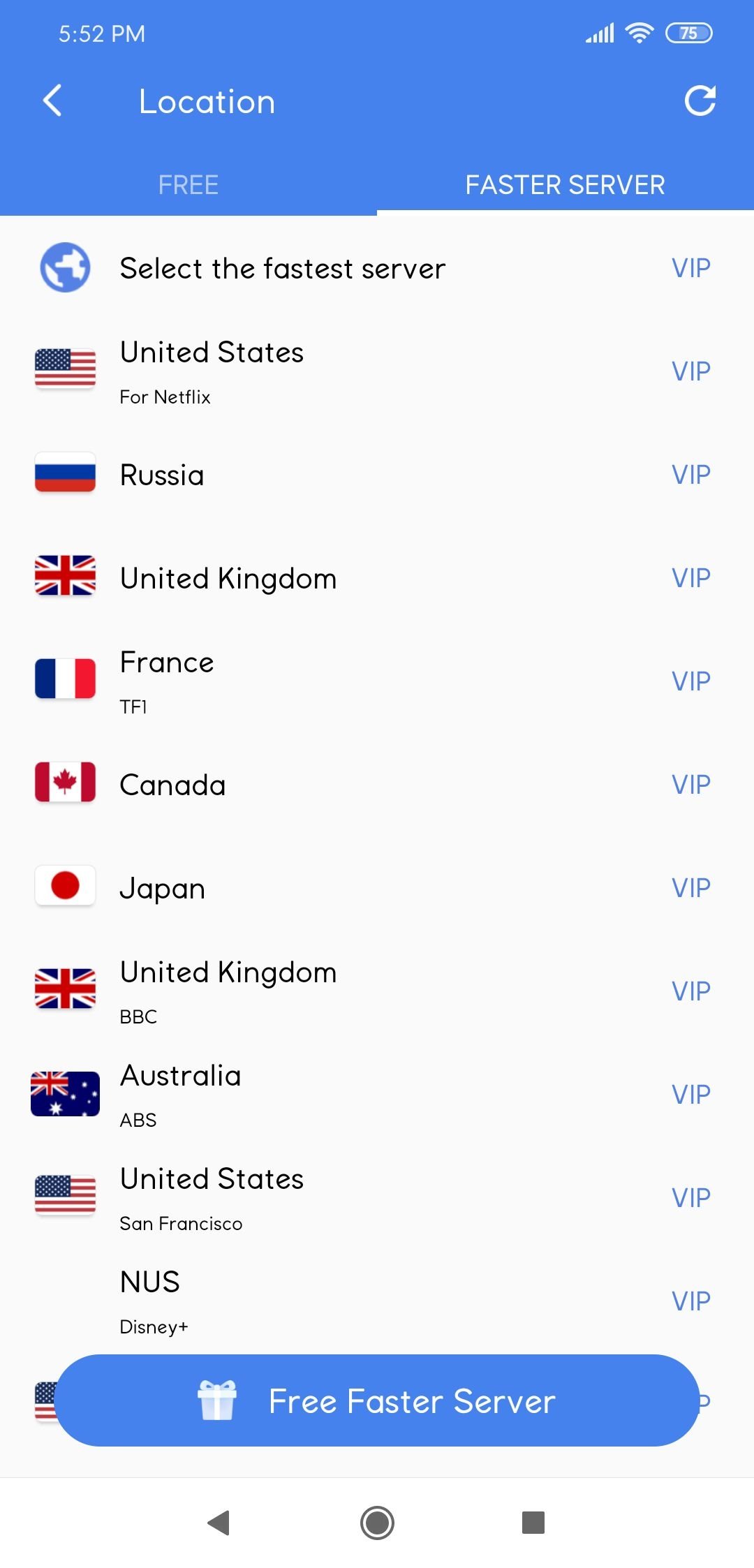The image is a screenshot of a smartphone displaying a website interface. The header is a stunning sky blue color, featuring elements in white font. Positioned on the upper left corner, it indicates the time: "5:52 p.m." On the upper right corner, there is a battery icon showing a 75% charge level.

Beneath the header, a section labeled "Location" is displayed in white, with the word "Free" situated below it. Adjacent to this, on the right, it reads "Faster Server." 

The main content area presents a list of various countries, each accompanied by its national flag on the left and tagged as "VIP" on the right. The countries, ordered from top to bottom, are as follows:
- United States (Stars and Stripes flag)
- Russia
- United Kingdom
- France
- Canada
- Japan
- United Kingdom (with "BBC" noted underneath)
- Australia
- United States (with "San Francisco" noted underneath)

At the very bottom of the screen, there is a rectangular button with rounded corners, also in the enchanting sky blue color. The button has the text "Free Faster Server" written in white, and to the left of this text, there is a small icon resembling a gift package.